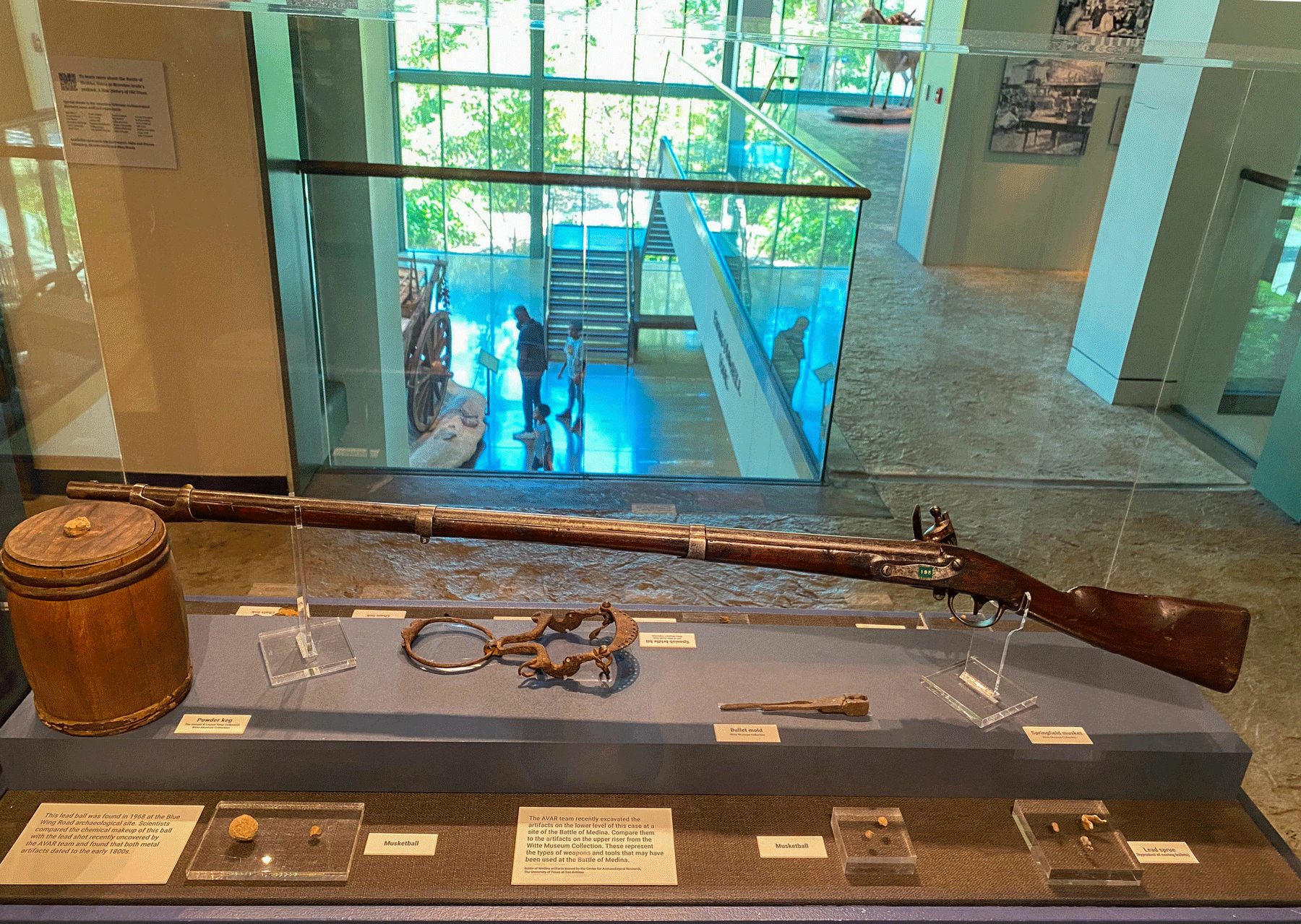The photograph captures a detailed indoor exhibit scene from a museum, showcasing an old-fashioned 18th-century front-loading, muzzle-loading musket. The musket, which has a long and narrow design with a glossy, dark brown wooden stock and a dulled silver barrel, is displayed inside a glass exhibit case. The gun is oriented with its barrel pointing to the left and its butt on the right side, highlighting its intricate features such as the metal trigger guard and the flintlock mechanism on top. Sitting to the left of the musket within the display case is a light brown keg. In front of the case, a wooden shelf holds several flat display cases containing embedded small objects, each accompanied by white description placards. Surrounding the area, the museum features floor-to-ceiling glass walls, through which a lower floor with people standing by a stairway is visible. The indoor exhibit area has beige walls adorned with more artifacts and frames, and glass barriers are strategically placed around the exhibits. Visitors can be seen walking around, engaging with various displays, enhancing the vibrant atmosphere of the museum.